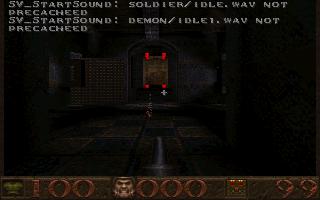The screenshot captures a scene from the video game Quake, highlighting the interface and some technical issues. Dominating the upper portion of the screen, white text reads "5e start sound soldier.idle.wave not pre-cached, sv start sound demon.idle.wave not pre-cached," indicating sound errors due to insufficient video card support. The dark room, primarily featuring brown and black tiles, forms the background. At the bottom, a horizontal status bar displays crucial player information: on the left, a green armor icon with a red "100" number, a human head with "000" indicating god mode status, and a shotgun icon with "99" ammunition in red. This arrangement is accompanied by a health bar and ammunition count, essential for gameplay. Centrally positioned on the floor amid the tile-based design is a brown box framed by bright red clips, resembling a picture frame. The overall scene is shrouded in darkness with occasional gray elements, enhancing the ominous setting typical of Quake.